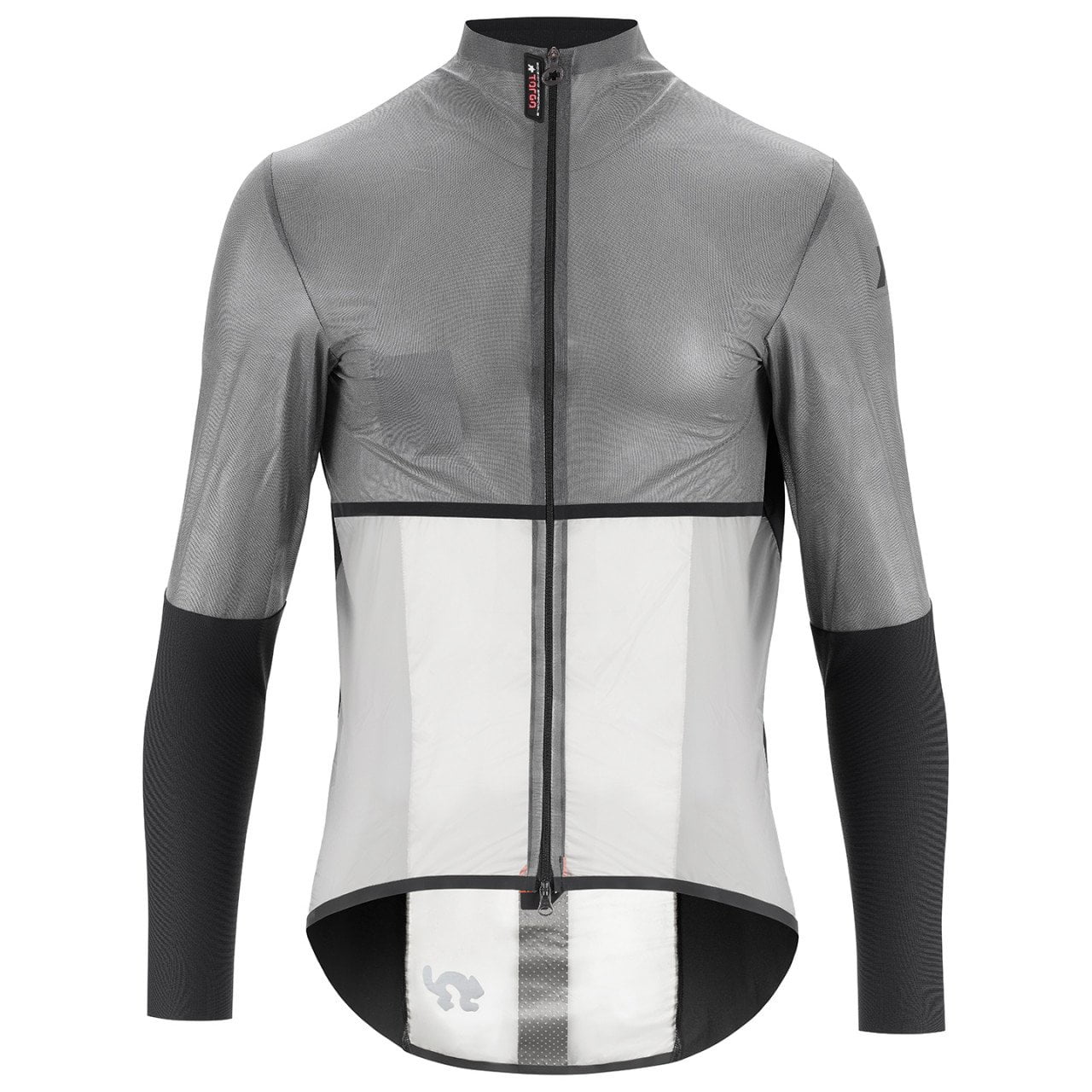The image depicts a sleek, multi-tone running jacket designed for athletic use, displayed against a white background. The jacket features a full-length black zipper that runs from the bottom to the collar, which envelops the lower portion of the neck. The upper half, including the area from the mid-ribs up and the chest, is a light silver-gray. The lower part of the body down to the abdomen is primarily white with some gray stripes on the sides and a gray line running along the zipper. The forearms, extending from the elbows to the wrists, are a solid black. The fabric appears thin and form-fitting, ideal for activities like running or cycling. A small pocket is present on the left-hand breast from the wearer's perspective, and a tag with red writing, partially visible and bearing letters "T-O-R-A-N," hangs from the top. There's also an insignia on the left shoulder, though its details are unclear. The inner fold mirrors the outer stripes, adding a reflective quality. The front of the jacket is higher than the back, adding to its aerodynamic design.